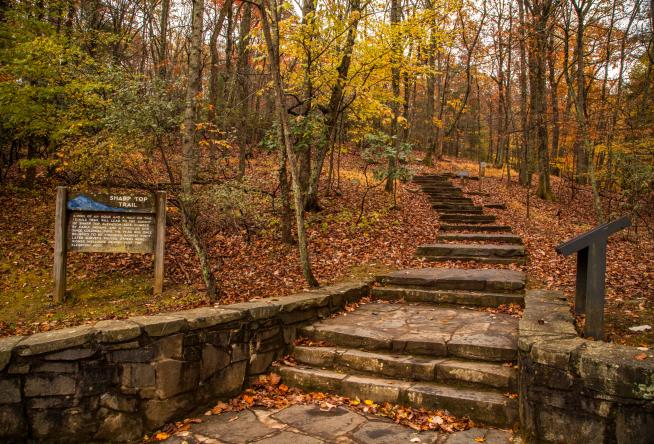This is a detailed photograph capturing the entrance of the Sharp Top Trail in a park. Taken from the bottom of cobblestone steps, the trail ascends diagonally to the upper right, with steps zigzagging through a forest adorned in vibrant autumn colors. On the left side of the image, there is a brown fence post with a wooden sign indicating "Sharp Top Trail." The cobblestone staircase is bordered by a retaining wall made of similar stones. The ground is carpeted with a mix of brown, red, and yellow fallen leaves, indicative of the fall season. The trees in the background exhibit a beautiful spectrum of autumn foliage, with leaves in shades of yellow, red, and some lingering green. A glimpse of another sign made from black wood can be seen on the far right, though its text is not visible. The setting is captured during daylight, offering a clear, inviting pathway into the forest.